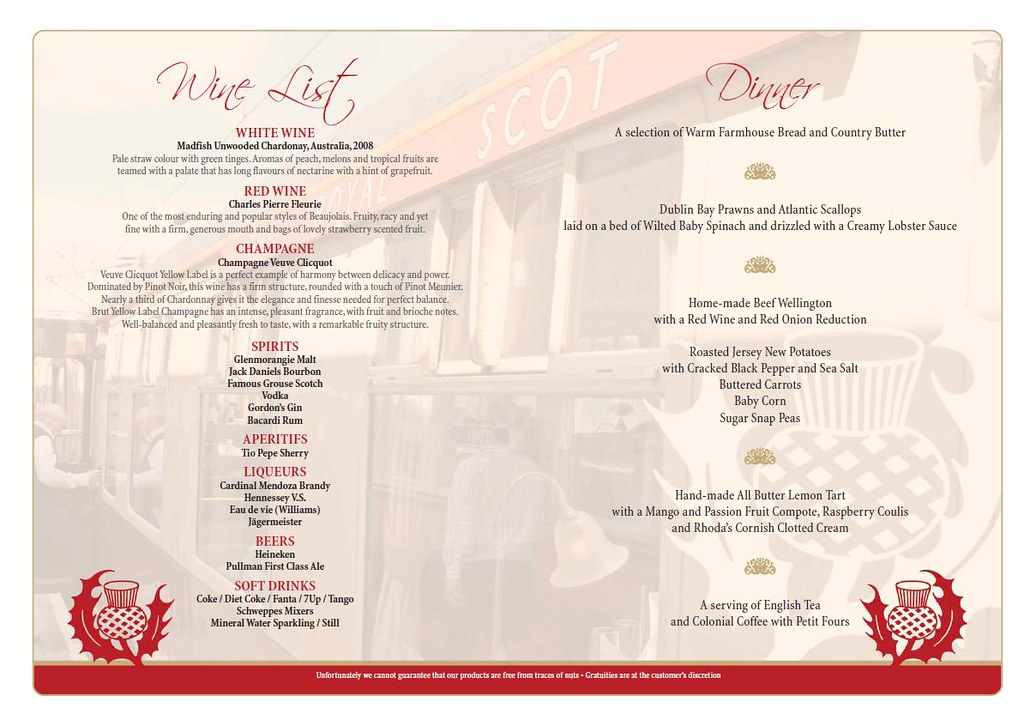The image showcases a horizontal rectangular menu with a blurred light beige and pink-red background featuring the front of a building, likely a restaurant named "Royal Scott," indicated by an orange banner at the top. The menu is divided into two sections. On the left, the "Wine List" is prominently displayed in red, featuring categories like white wine, red wine, champagne, spirits, liqueurs, beers, and soft drinks. On the right is the "Dinner" section, which offers a detailed formal dining experience. The menu lists a selection of warm farmhouse bread and country butter, Dublin Bay prawns, Atlantic scallops on a bed of wilted baby spinach with a creamy lobster sauce, homemade beef Wellington with a red wine and red onion reduction, roasted Jersey new potatoes with cracked black pepper and sea salt, buttered carrots, baby corn, sugar snap peas, a handmade all-butter lemon tart with a mango passionfruit compote, and Cornish clotted cream. The meal is rounded off with English tea and colonial coffee served with petit fours. Both sides of the menu feature a red line at the bottom and a logo that depicts a red leaf inside a bottle, using predominant colors of red and white.